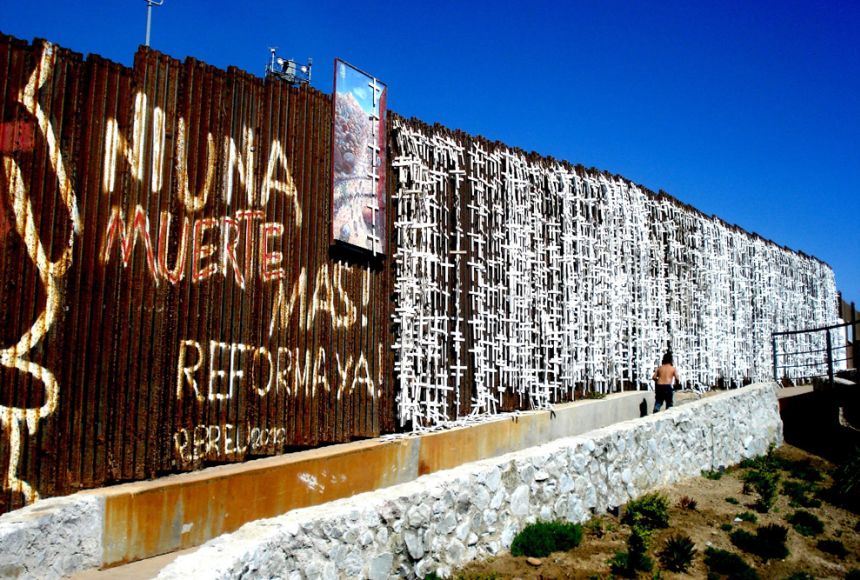The photograph captures an extensive outdoor wall composed of rusted, corrugated metal with a white-painted surface and a concrete foundation. The top is adorned with barbed wire and some lighting fixtures. The wall prominently features graffiti text in Spanish, including "Ni Una Muerte Más Reforma Ya!" White wooden crosses adorn the metal surface, extending across the length of the fence as a poignant memorial, possibly indicating numerous deaths, perhaps in relation to border crossings. Nearby, a stone wall built from white stones runs along the concrete walkway, which also features metal railings and a concrete stairway. In the image's upper right, a clear, cloudless blue sky provides a serene backdrop. A shirtless man in dark pants is walking along the path away from the camera, near where the stone wall ramps up. The area surrounding the wall is mostly devoid of grass, emphasizing the stark and somber atmosphere.